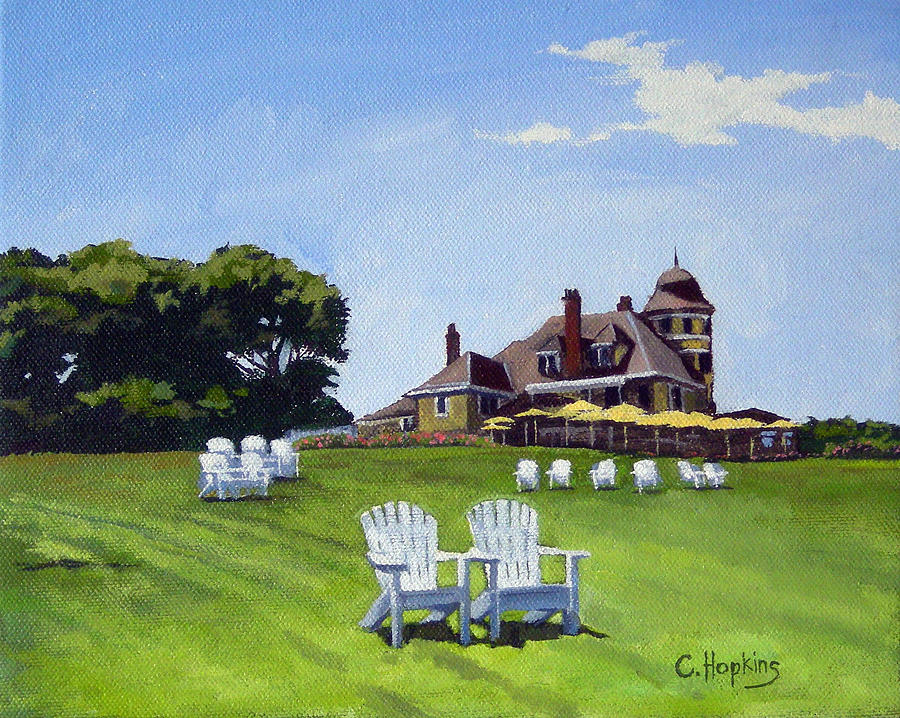The painting, created by C. Hopkins, captures a serene outdoor scene that evokes the calm ambiance of locales like Cape Cod or Hyannis Port. The foreground is dominated by a lush, expansive green lawn scattered with white wooden Adirondack chairs, including two prominently positioned at the very front. An organized arrangement of six chairs lines the right side, while more chairs are situated up to the left. 

The backdrop features a grand Victorian-style house, painted in a deep yellow hue with a brown roof and several brown chimneys. The house appears to have two main stories and a three-story tower behind it. In front of the house, a series of yellow outdoor umbrellas suggest the presence of tables and chairs beneath them, further hinting that the location could potentially be a restaurant or a gathering place. Tall trees flank the house, with some large trees prominently on the left and additional trees appearing in the background to the right. Above this tranquil setting, the sky is a bright blue dotted with a few puffy clouds, enhancing the peaceful and picturesque atmosphere of the scene.